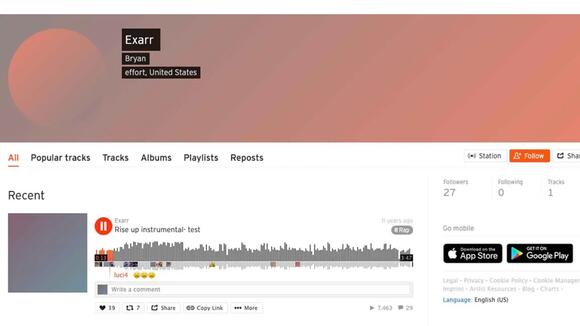This is a color photo depicting a website interface, possibly a music or podcast platform. The image appears small, even when magnified to 100%, making the text difficult to read. Dominating the top of the page is a large orange band with white space above it. On the left side of this orange band, there is a shadowy outline of the sun, shaded with grey.

To the right of this sun icon, the interface features white text on black squares, displaying terms like "EXARR," "BRYAN," and "EFFORT, United States." This section seems to showcase a playlist or podcast information. Below this, several red tabs are aligned to the left, labeled "Popular tracks," "Tracks," "Albums," "Playlists," and "Reposts."

Adjacent to these tabs, there are options in an orange font, including "STATION" and "FOLLOW," accompanied by "SHARE" in a different section. Directly below is a category labeled "RECENT," with a grey square featuring a graphical representation, possibly denoting a track.

Within this grey square, there is a red circle, a STOP button, and text reading "RISE UP INSTRUMENTAL TEST." A comment box beneath this invites user interaction with the prompt "WRITE A COMMENT."

Further to the right, user engagement metrics are displayed, showing "FOLLOWERS 27," "FOLLOWING 0," and "TRACKS 1." Additional instructions encourage users to "GO MOBILE" by downloading the app from the Apple Store or Google Play. The language setting, "ENGLISH US," is also visible, although some elements are too greyed out to decipher. The overall impression suggests the website features an album track or podcast.